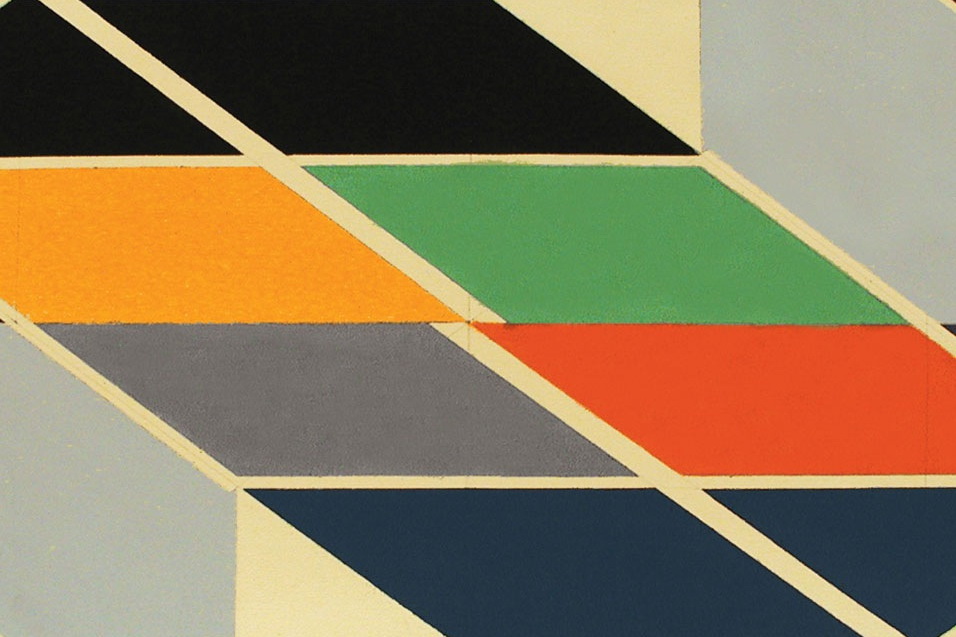The image features a bright geometric pattern composed of various colored squares arranged diagonally. Starting from the top left corner, two black squares are separated by a beige stripe. Below them is an orange square, which is also divided by the same beige stripe, leading to a green square. Continuing downward, a red square is situated with a lavender square to its left. At the lowest part of the image, two navy blue squares appear, each separated by the recurring beige stripe.

In addition to the central squares, the pattern includes a distinct structure of lines. On the left-hand side, a brownish line runs vertically, splitting into a road-like formation that is two cubes wide. This line breaks off about halfway up, creating an inch-long separation where the cube corners touch, before continuing to the base.

The sides and perimeters of the cubes showcase different colors: the side facing the viewer alternates between a darkish gray and a yellow side for the bottom row. Behind this arrangement, there is a gray wall, while the topmost edge of the pattern is framed by a yellow wall, seamlessly blending with the geometric design. The framing lines of the image are beige, matching the stripe and forming a beige triangle in the right-hand corner.